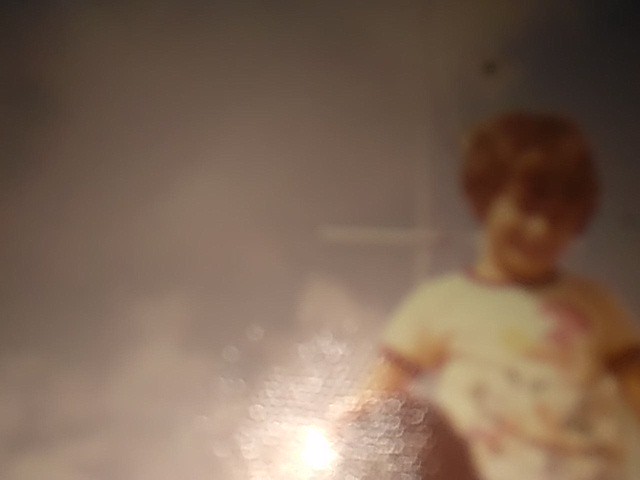A blurred and faded vintage photograph reminiscent of color photos from the 1950s through the 1970s. The image features a child with short brown hair that covers the ears, making it difficult to determine the gender. The child has a visible, though indistinct, smile, and you can barely discern their nose and eyes. They are wearing a short-sleeved t-shirt with a crew neck that has a dark-colored band. An unclear design is printed on the shirt. The majority of the background is gray, with darker gray corners and a rose-gray center. To the right of the child, there's a bright white light, possibly from a bike, emanating from their right arm area, surrounded by small lens flares.